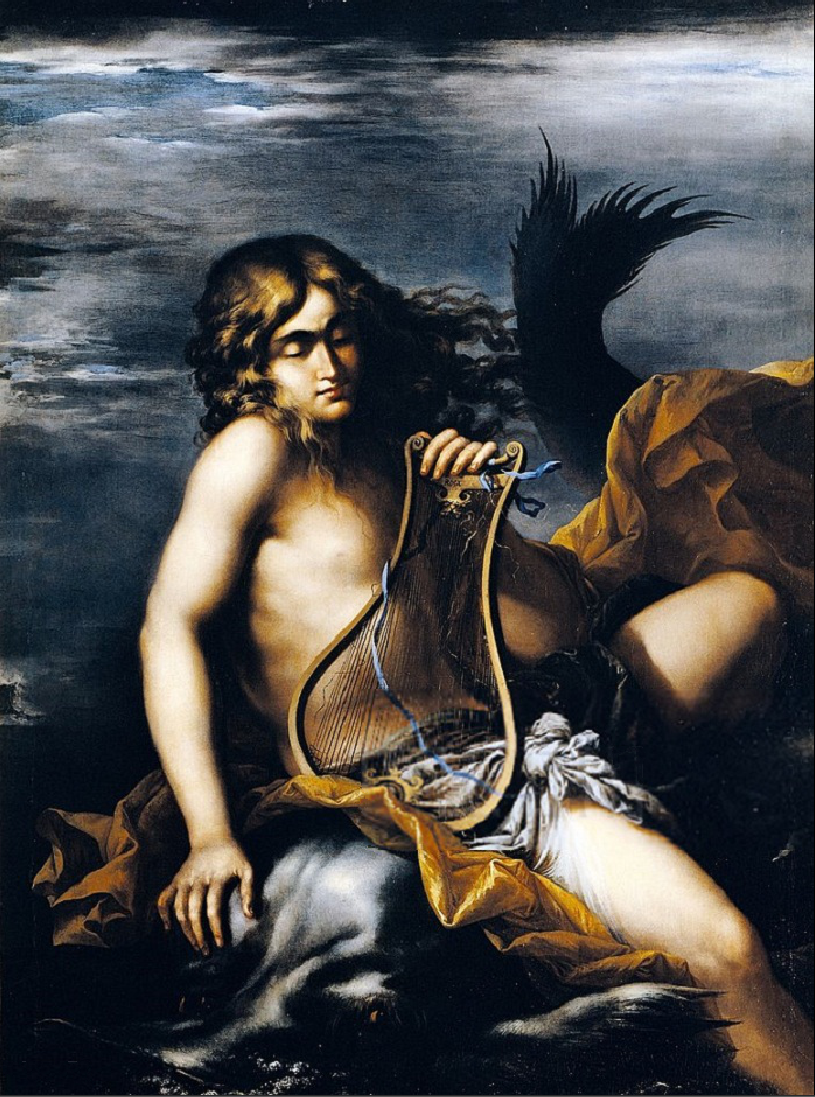This detailed painting, evocative of a Baroque or Rembrandt style with its dramatic interplay of light and shadow, features a young male figure as its central focus. The individual, possibly a boy, has long, curly brown hair that flows to the right of his face, giving the impression of movement as if stirred by a breeze. Set against a dark blue and black background, the ambiguity of sky or water adds to the enigmatic atmosphere of the image.

Seated slightly angled to the right, the figure's chest is bare, with yellow-gold and dark yellow fabric—perhaps robes or towels—draped across his waist and extending beneath him. His legs are slightly separated as he sits. His left hand gently rests on a small, stringed musical instrument resembling a harp, while his right hand is positioned on the fabric beside him. His downward gaze suggests contemplation or focus on something below.

Adding to the painting's mystique, there is a large black form adjacent to the right of the fabric, and a paw-like shape with pronounced claws near the figure's right leg, though its source is obscured. Dominated by flesh tones, the color palette also incorporates shades of blue and gray, further deepening the sense of depth and drama in the scene.